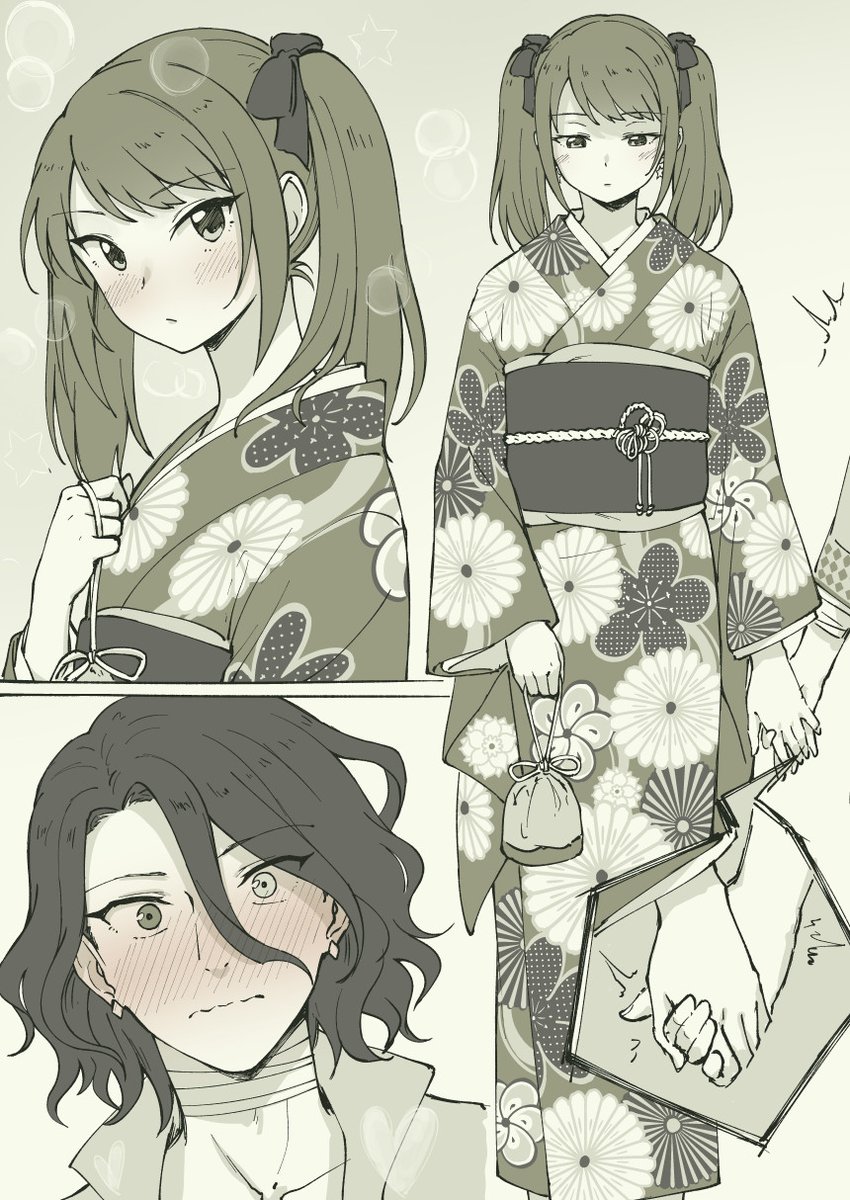The rectangular, black-and-white manga drawing, taller than it is wide, showcases three distinct scenes involving two young women. In the upper left portion, there's a close-up of an Asian girl with light skin, adorned in a floral yukata. Her body is turned to the left, revealing her from mid-bicep upwards, her face gazing back at the viewer over her shoulder with a subtle blush on her cheeks. Her hair is styled in ponytails. 

On the right half, the same young woman is depicted standing almost from her feet upwards. She wears the same floral yukata with a large waistband, her head tilted down and a blush adorning her cheeks, a neutral expression on her face. Her hands are at her sides, except in an insert towards the lower right side of this section, where she is seen holding the hand of someone next to her. A speech bubble emanates from the hand-holding scene.

In the bottom left corner, there's a separate box featuring another young woman with curly, shoulder-length black hair. She is wearing an open-collared jacket, her eyes wide open in a startled expression, mouth slightly frowning, with pronounced blush lines across her face. Her eyes are distinct, one green and the other light blue, and she has heavy eyeliner on, contributing to her shocked demeanor.